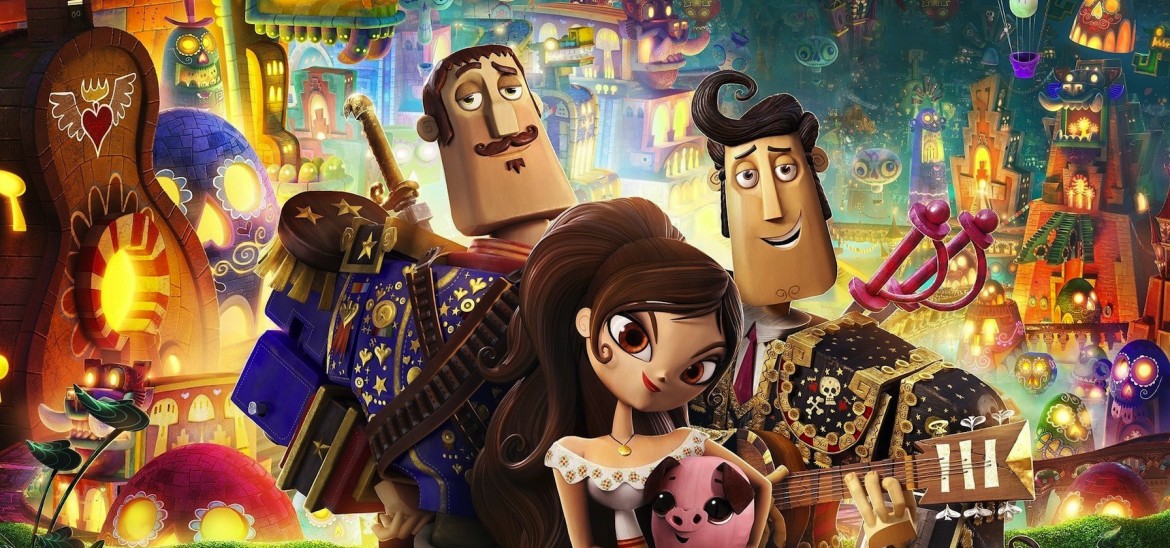The vibrant animated scene resembles a Pixar movie preview. It features three central characters: a charismatic man with a pompadour hairstyle reminiscent of Elvis, strumming a guitar; another man beside him in ornate, mariachi-like attire, wielding two swords; and a smiling woman with dark hair, dressed in a white off-the-shoulder shirt, cradling a baby piglet. Together, they stand against a festive and bustling backdrop that evokes a carnival or Halloween atmosphere, full of colorful lights and animated details. The background is adorned with glowing skull-like lanterns, robotic figures with lit-up eyes, and a rich palette of yellows, oranges, blues, and purples, creating a lively and enchanting visual feast.